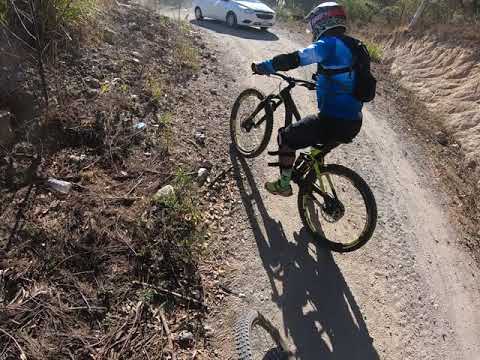The photo captures an outdoor scene in the mountains where a young person, seemingly an early teen, is riding a black mountain bike with bright green or yellow accents. The rider is dressed in a blue long-sleeve windbreaker and black pants, complemented by green shoes and yellow socks. They are equipped with a white helmet featuring a red strap, a backpack, and protective pads on their arms and legs. The person is seen steadying themselves on a gravel roadway with their right foot on the ground and left foot on the pedal, indicating a pause while navigating the steep, hilly terrain. Flanking the gravel road are patches of grass mixed with dirt. In the distance, a white sedan is approaching from the opposite direction, partially cut off at the top of the image, adding to the dynamic and adventurous atmosphere of the scene.